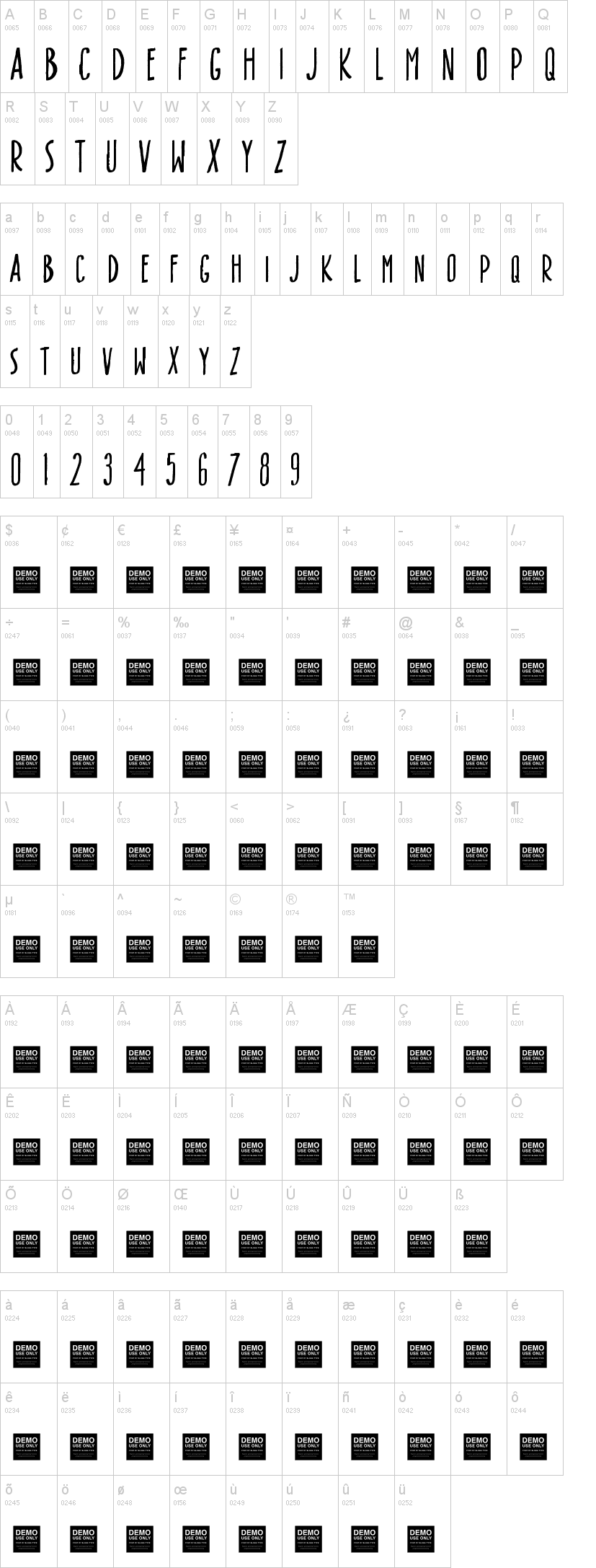The image depicts a unique, keyboard-like layout designed to resemble a piano keyboard with shaded black sections. At the very top, there is a sequence of uppercase letters from A to Z, each accompanied by numbers starting from 0065 and ending at 0090. These uppercase letters are all in black.

Below this section, there's a line of the alphabet in lowercase letters, also from A to Z, with corresponding numbers starting from 0097 and ending at 0122. Beneath this row is a repetition of the uppercase alphabet in black. 

Additionally, there is a numeric section at the bottom, ranging from 0 to 9 with numbers starting from 0048 and ending at 0057. Scattered throughout the layout are various symbols, including dollar signs and other common keyboard characters, suggesting it could be similar to a cell phone keyboard. 

A notable feature of the layout is the label "DEMO USE ONLY" prominently displayed in a black box.